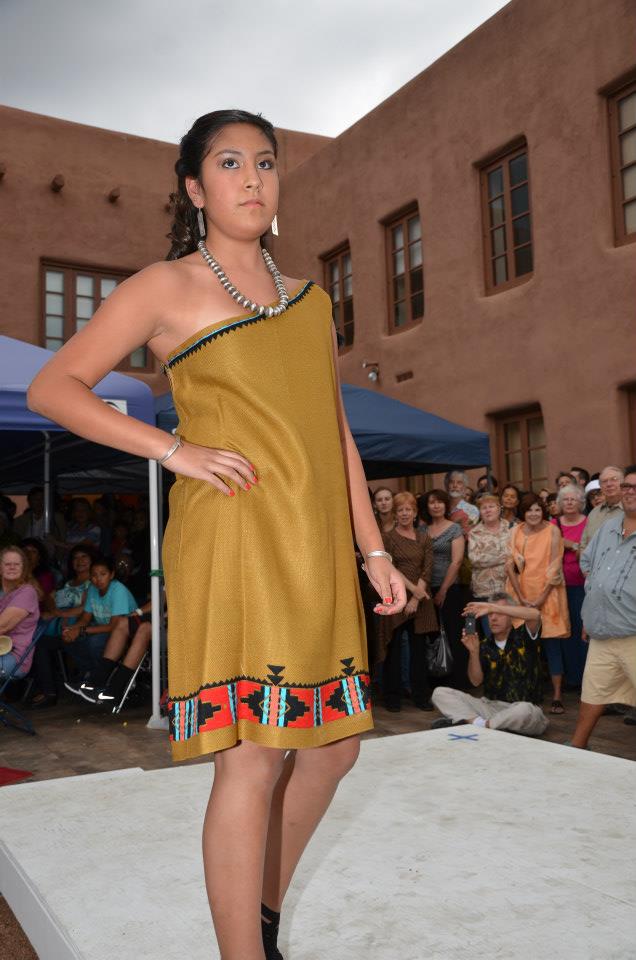In this color photograph, a young lady, approximately 17 years old, is seen modeling a Native American-inspired dress at an outdoor event, possibly a fashion show. The setting is a courtyard framed by red adobe-style buildings. The image is in portrait orientation, showing the model from head to ankles. She stands on a white platform with one hand on her hip, facing the right side of the image while looking slightly upward. Her long, dark black hair is pulled back, accentuating her distinctive silver dangly earrings and a silver beaded necklace.

The dress she is modeling is made of gold fabric with a one-shoulder design, adorned with a black zigzag trim near the neck. The bottom of the dress features a horizontal band with Native American-inspired patterns in orange and aqua, highlighted by black triangles. The dress extends to just above her ankles, crafted in a shift style. 

A decent-sized crowd is visible behind her, attentively watching the fashion presentation. Additionally, a man sitting cross-legged on the ground to her right points a camera towards her. The image captures the realism and representationalism of fashion photography, emphasizing the cultural and stylistic details of the attire.